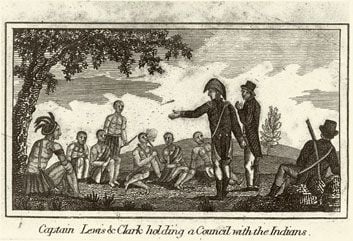The image is an old black-and-white sketch on yellowed paper, measuring approximately two inches wide and an inch and a half high. The bottom of the image is labeled in black print, "Captain Lewis and Clark holding a council with the Indians." The sketch is bordered by a thin pinstripe, enclosed within a lighter pinstripe border. The scene depicts a historic council meeting, likely from the early 19th century. 

On the right side stand Captain Lewis and Clark, adorned in long-tailed jackets, light-colored pants, boots, and hats. One of them extends his left hand, while the other clasps both hands as they engage in conversation. Among them, a man is seated on the ground holding what appears to be a gun. To the left, a group of Native Americans forms a semicircle, most of them seated except for one individual standing. A tribal chief is distinguished by his position under a tree on the left. Above the group, the sky is sketched with faint clouds, adding depth to this evocative scene of early American history.